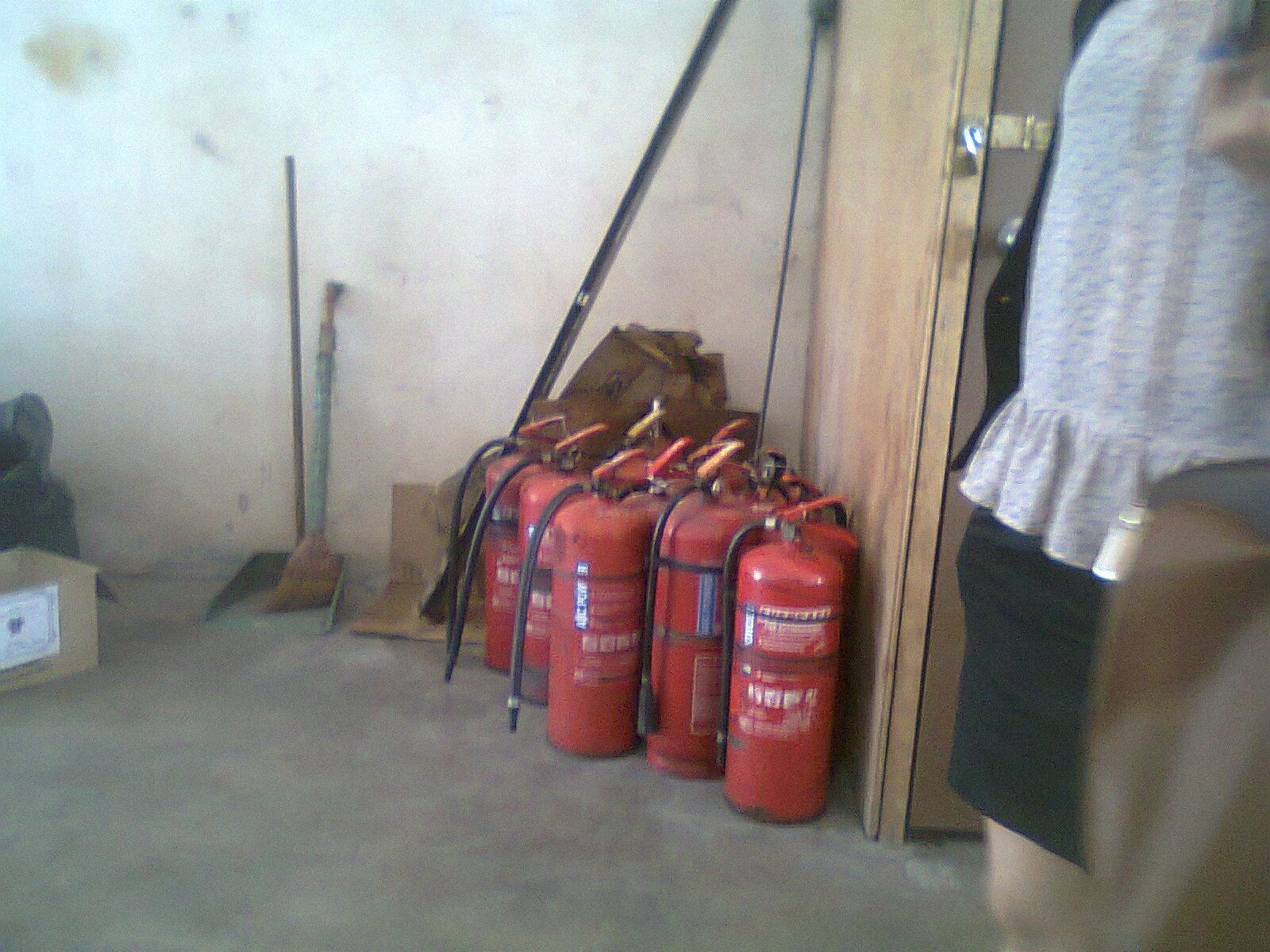In the image, the scene is set inside a storage room with bare cement floors and unpainted, slightly dirty white walls. Dominating the center of the image is a collection of red, commercial-sized fire extinguishers, numbering between seven and nine, propped up next to the wall. Each extinguisher has black rubber hoses and visible nozzles, indicating they are ready for use, though they appear dirty and possibly old. To the right of the extinguishers, there is a cleaning set comprising a dustpan with a long handle and a short, well-used broom. The dustpan's handle is notably taller than the broom. On the left side of the image, a box with white text can be seen, while to the right, some folded-up cardboard leans casually against the wall. Additionally, a person stands partially visible on the far right, wearing a white patterned blouse, black skirt, and holding a brown bag. The visible part of this person extends from the neck to the knees. There are also small black holes noticeable at the top right and bottom right corners of the image, adding to the room's rugged appearance.